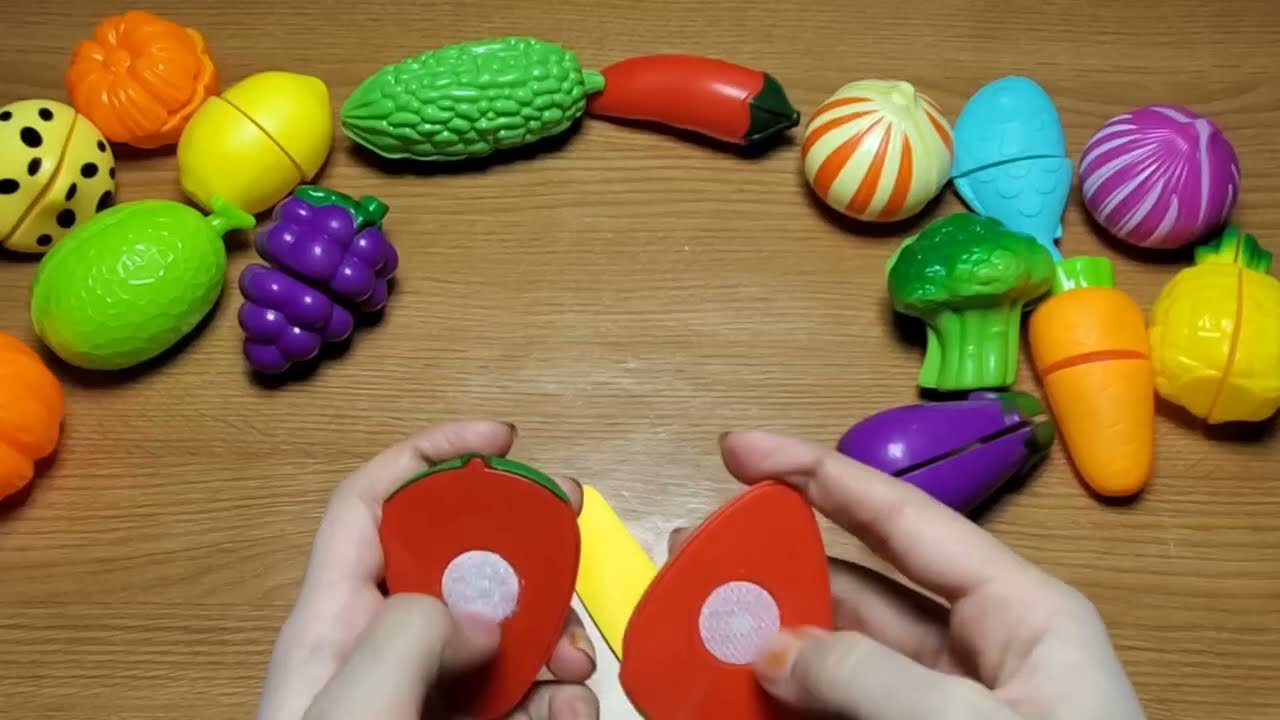The photo showcases a light-skinned person’s hands holding a pair of plastic strawberries, each about half the size of the person's palm. The strawberries are split down the center, revealing two white circular Velcro pads, one of the sticky side and the other fluffy. The background features an array of colorful plastic fruits and vegetables meticulously spread out on a wooden table. This collection includes a segmented orange carrot, green corn, purple grapes, a purple onion, an orange and white onion, a red pepper, a green lime, a squash, and an orange pumpkin. Other visible pieces are broccoli, a lemon, an eggplant, a pear, and a pineapple. All the fruits and vegetables are vibrant in colors ranging from yellow to blue and are designed to split in half, highlighting their toy-like nature. The scene suggests that the individual is organizing or playing with these detachable toy produce items, possibly as part of a demonstration or a sorting activity.